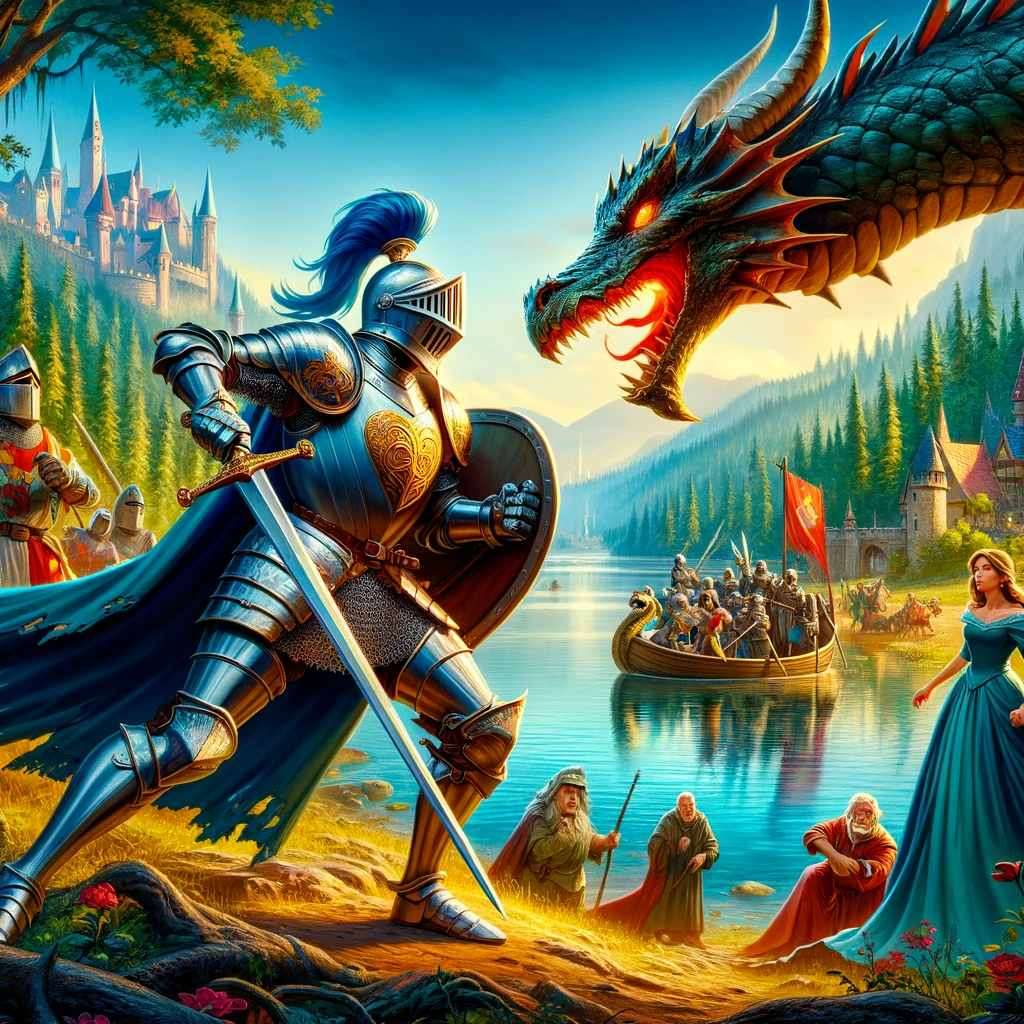In this vivid and fantastical scene bathed in afternoon sunlight, a brave knight, clad in gleaming silver armor with a striking blue plume on his helmet, stands resolutely on a cliffside, ready to confront a menacing dragon whose fiery eyes and dual tongues add an air of imminent danger. The dragon, emerging from the right, locks eyes with the knight, its dark scales contrasting sharply with its glowing red eyes and mouth. The knight, marked by a golden heart emblazoned on his chest, grips a towering sword and a stout shield, poised for battle.

To the left, perched atop a rugged cliff, a medieval castle looms over the tableau, partially obscured by a tree. Below, at the water’s edge, several peasants and a noble maiden in a flowing blue dress watch the impending clash in awe. Greenery sporadically dots the landscape, adding life to the mythical setting. Meanwhile, three additional knights, distinguishable by their red sashes, stand vigilantly nearby, forming a protective cadre around the scene.

Further back, a ship brimming with more knights sails swiftly across the lake, poised to lend their aid. The tableau blends elements of high fantasy with vibrant, cartoonish colors, creating a rich, computer-generated art piece laden with anticipation and epic grandeur.